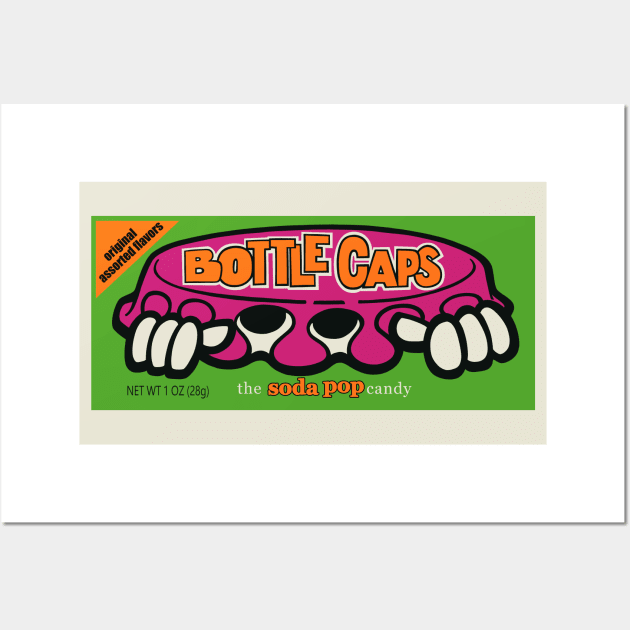The image depicts the vibrant advertisement for a candy company called "Bottle Caps." Central to the image is a dynamic, anthropomorphized pink bottle cap character, complete with large, whimsical googly eyes and white hands jutting out from its sides. The character seems lively and engaging. Above the character, the name "Bottle Caps" is prominently displayed in orange text. The main background of the image is a bright green, contributing to the eye-catching design.

In the top left corner, an orange triangle bears the text "Original Assorted Flavours." At the bottom of the green rectangle, the product is labeled "The Soda Pop Candy," with "Soda Pop" highlighted in orange text. The weight information, "NET WT 1 OZ (28g)," is provided in black text.

Surrounding this central green rectangle, the image layers several borders: a light gray or beige outer square, a white rectangular frame, and a light brown or beige inner rectangle, each adding depth to the overall design.